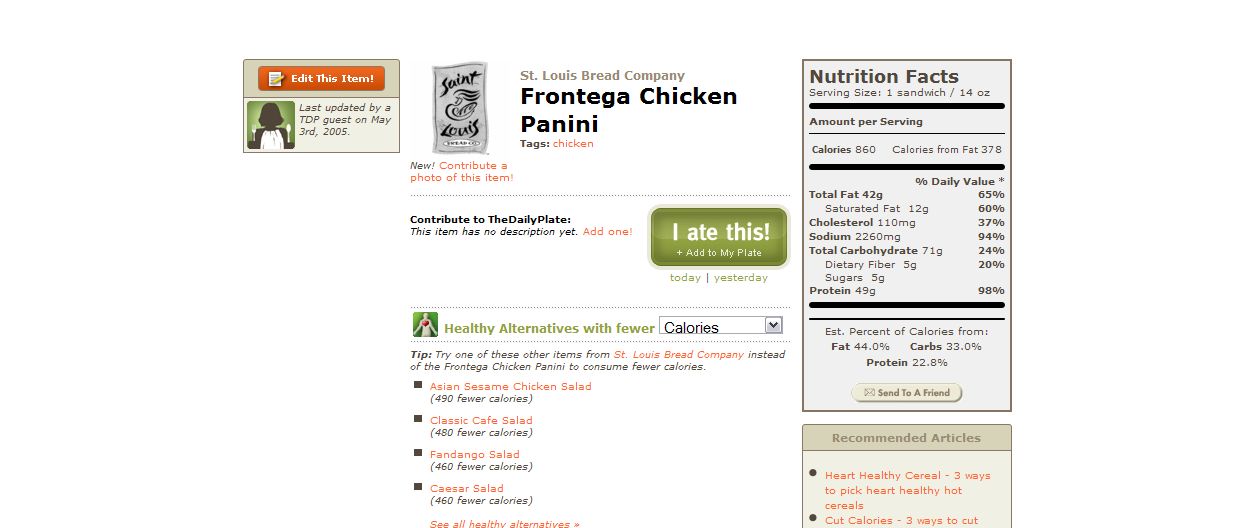The image appears to be a screenshot from a webpage with a white background, showcasing a food item named "Frontega Chicken Panini, St. Louis." Above the item name is text encouraging contributions to the daily plates. The panini itself lacks a detailed description on the page. To the left, there's a prominent green button labeled "I ate this," promoting it as a healthy alternative with fewer calories. On the right side of the image, a box displays the nutrition facts: 860 calories, 42 grams of fat (including 12 grams of saturated fat), 110 milligrams of cholesterol, 2,260 milligrams of sodium, 71 grams of total carbohydrates (with 5 grams of fiber and 5 grams of sugar), and 49 grams of protein.